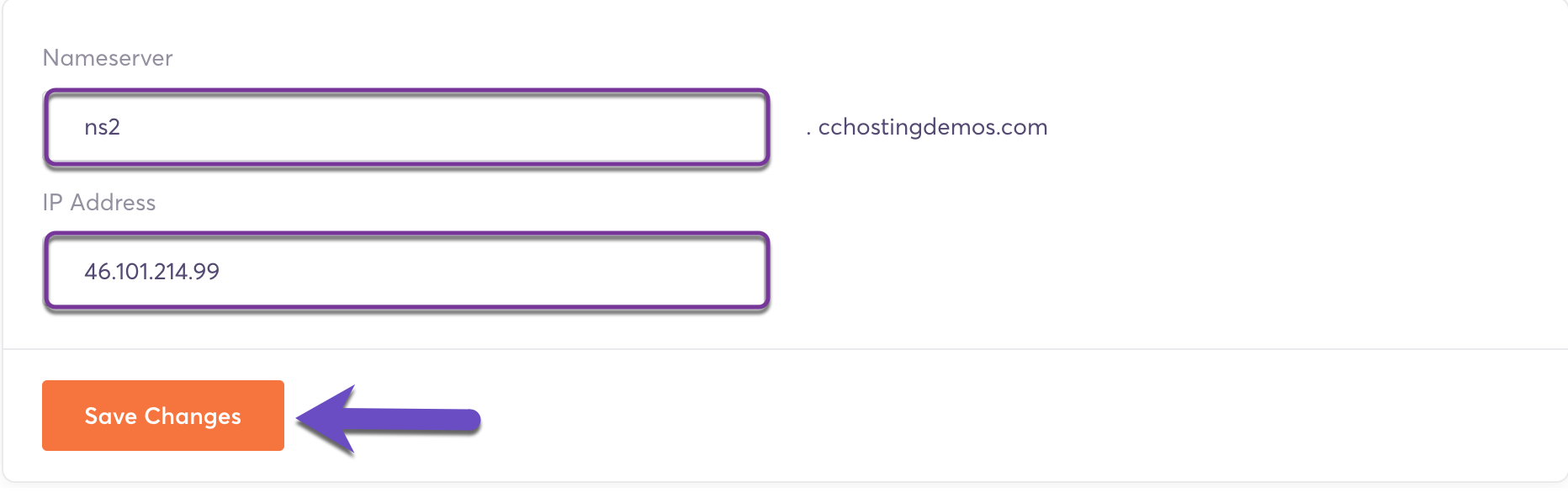The image is a narrow horizontal rectangle screenshot set against a white background, framed with a very thin gray line along the left and bottom edges. In the top left corner, the gray text "Name Server" is displayed. Directly below this label is a text field outlined in purple containing the text "NS2." To its right, the domain ".cchostingdemos.com" is shown. Moving left again, the label "IP Address" appears in gray, followed by another purple-outlined text field directly below, filled with the IP address "46.101.214.99."

Running parallel to the bottom border, a slender horizontal gray separator line divides the sections. Beneath this line, an orange "Save Changes" button is prominently situated. Adjacent to the button on the right, a horizontal purple arrow points leftward, directed towards the "Save Changes" button.